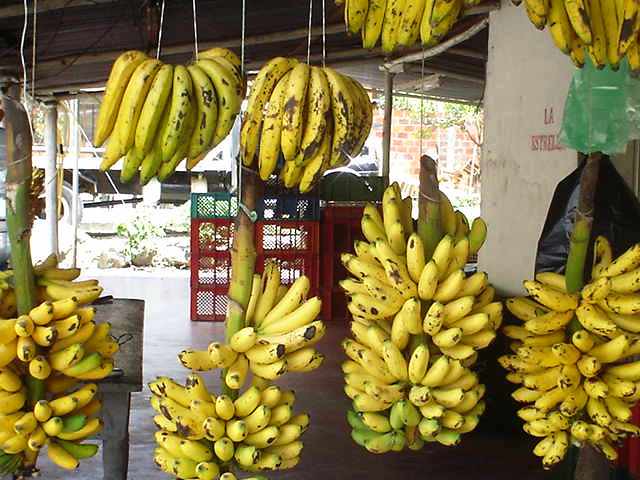This image showcases a bustling fruit stand at an outdoor market, with eight large bunches of bananas prominently displayed. The bananas, some still attached to their stalks, are suspended by wires or ropes with their ends curving upwards. They dominate the frame with their vibrant yellow color, speckled with dark brown spots, and some have hints of green. In the background, a white wall adorned with red lettering, possibly saying "La Estrella," is partially visible along with a stack of colorful milk crates in red, green, and black. On the left, a dark wooden table is seen, standing on a concrete floor. The market stall's structure is supported by thin metal poles, while the entrance features red and green metal doors through which sunlight spills into the scene. Beyond the shop, a large truck and brick buildings can be seen, adding depth to the lively marketplace atmosphere.